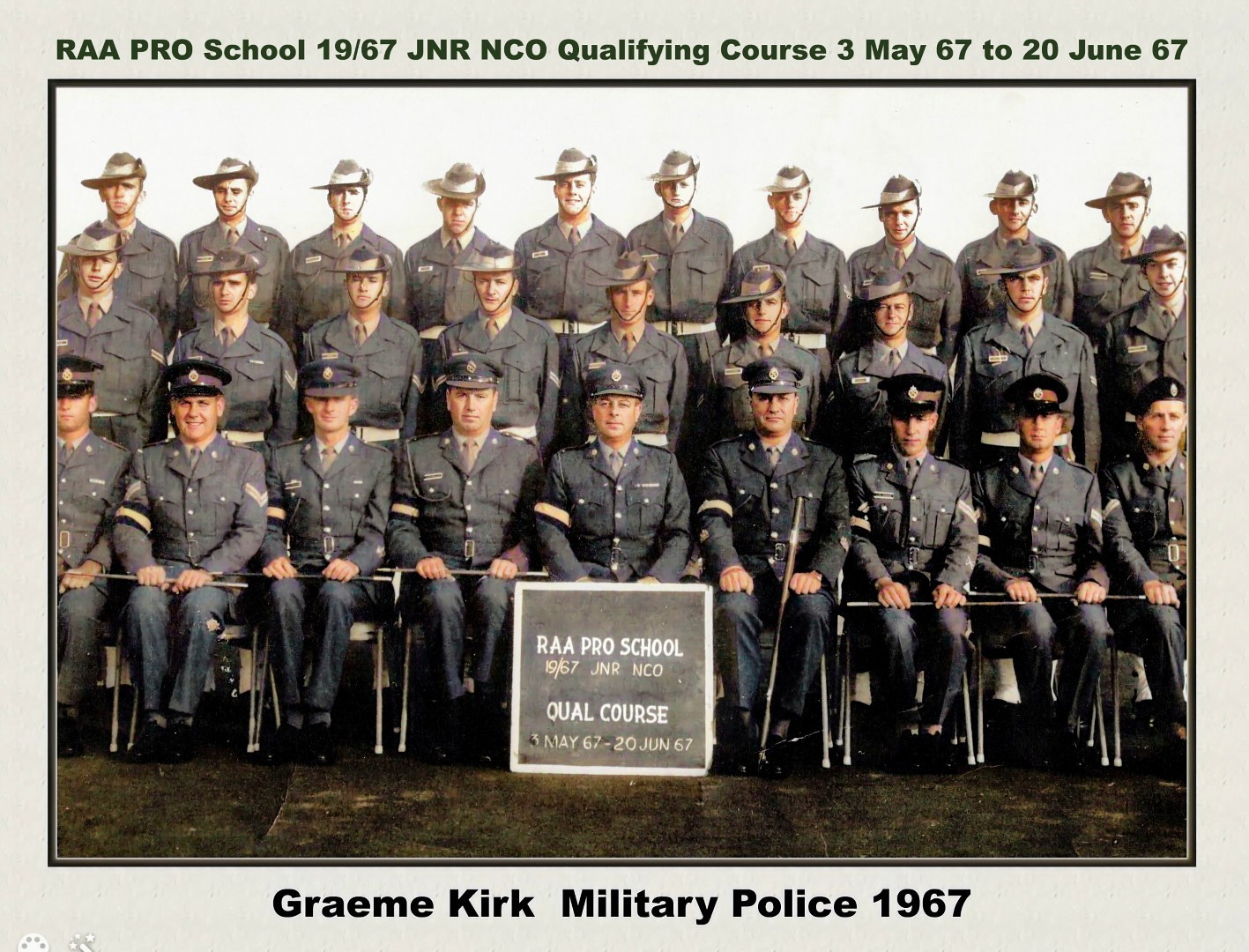This rectangular photograph, bordered in light gray, depicts a formal group portrait of military men from the RAA Pro School 1967 JNR NCO Qualifying Course, which took place from May 3, 1967, to June 20, 1967. The image shows a total of 28 men in three distinct rows. In the front row, nine men are seated in chairs, each holding a stick across their laps. They wear military uniforms that include gray coats buttoned up, name tags, and hats with a gold seal or badge. 

The second row consists of nine men standing, while the back row has ten men standing. Notably, the men in the front row wear flat-billed hats, giving them an officer-like appearance, whereas the men in the back rows sport more outdoorsy hats with chin straps, resembling cowboy hats. All individuals are dressed in full military attire. 

In the center of the front row is a blackboard sign that reads: "RAA Pro School 19/67 JNR NCO, Qual Course, 3 May 67 to 20 June 67." This same inscription appears in black font across the top border of the photograph. The bottom border reads "Graeme Kirk Military Police 1967," indicating the affiliation of the group.